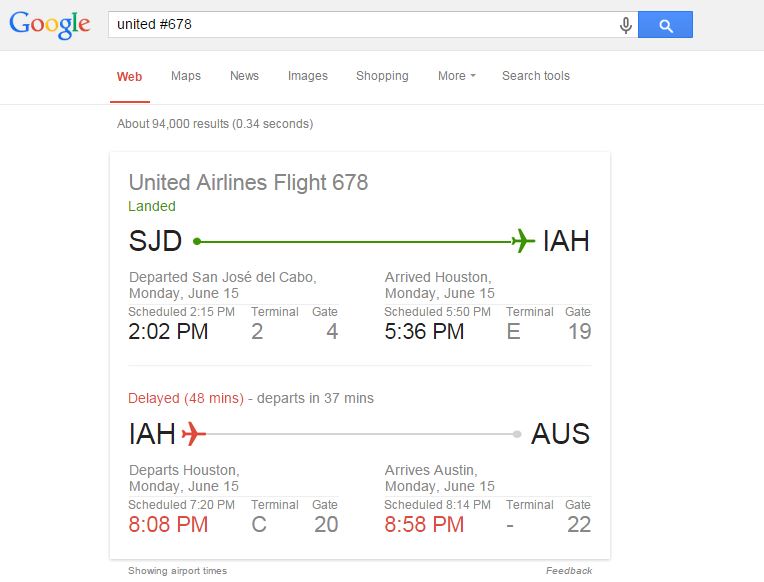A user searched for United Airlines flight 678 on the internet, yielding 94,000 results in just 0.34 seconds. The flight details reveal that United Airlines flight 678 departs from San Jose Del Cabo on Monday, June 15th, and arrives in Houston on the same day. The flight duration is approximately three hours and 15 minutes. However, it is delayed by 48 minutes and is scheduled to depart in 38 minutes. After landing in Houston, there is a subsequent flight to Austin, Texas, which is a 50-minute journey. There will be almost a three-hour layover before the departure for Austin, Texas, which is scheduled to leave at 8 PM.